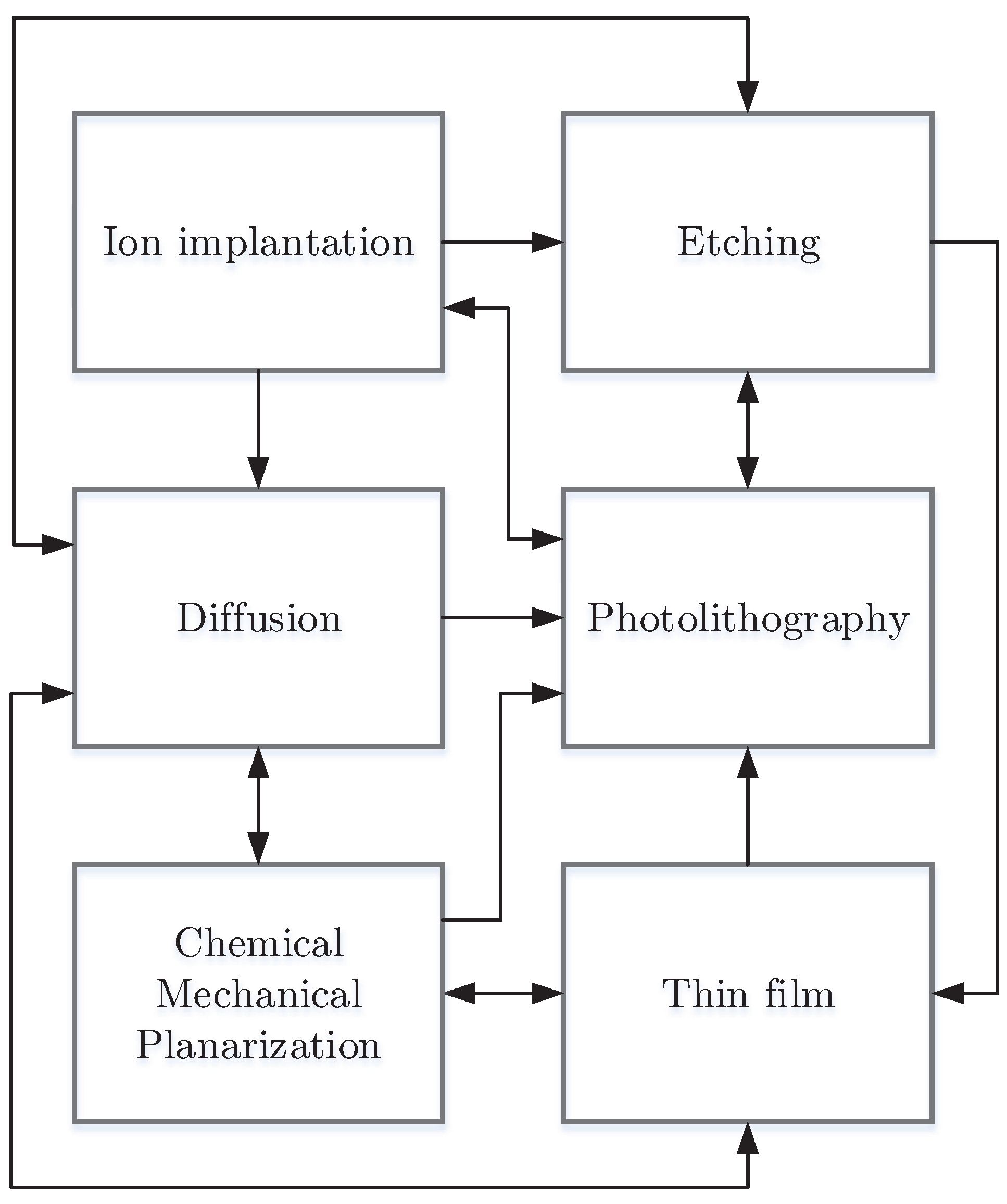A black and white flow diagram illustrating the complex, iterative process of making integrated circuits. The diagram consists of six interconnected boxes arranged in three rows of two, with numerous arrows indicating the flow between processes. Starting from the top left, the boxes are labeled as follows: "Ion Implantation," "Etching," "Diffusion," "Photolithography," "Chemical Mechanical Planarization," and "Thin Film." Each box is interconnected with black arrows, some unidirectional and others bidirectional, reflecting the repetitive and interconnected nature of chip manufacturing. The diagram is printed on a white background with black text and arrows, giving it a clean, scientific appearance reminiscent of educational materials found in science textbooks.